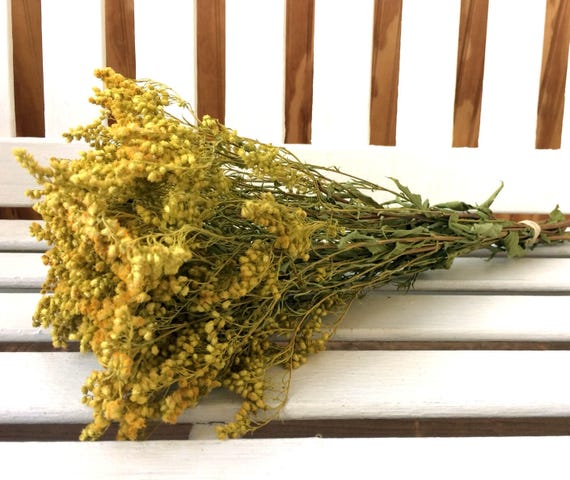The image features a dried bundle of yellow flowers laid on a white wooden bench. The stems, appearing brownish-green and withered, extend to the right, tied at the base with a light-colored rope or elastic band. The flowers, clustered on the left, resemble small yellow balls rather than open blooms. The background showcases a wooden wall interspersed with white sections. The photograph presents a top-down view, allowing the details of the bench and the tied bouquet to be clearly visible. Some leaves appear crumpled, accentuating the dried and aged nature of the bouquet.